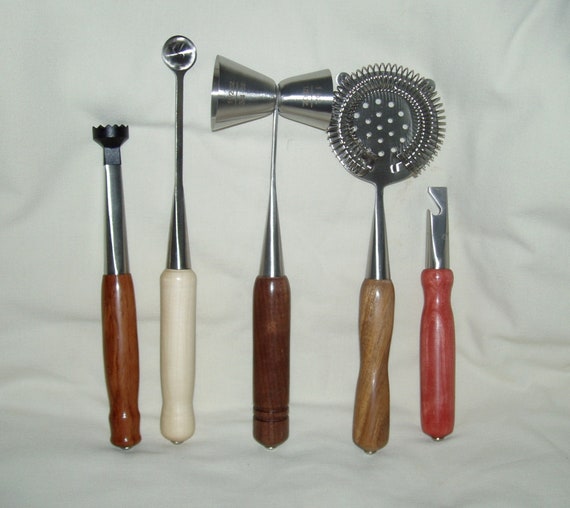The image depicts five bartending tools arranged on a white cloth background. Each tool features a uniquely colored wooden handle and a specific functional metal component. 

Starting from the left, the first tool has a medium brown, mahogany-looking handle and a silver tube ending in a black serrated tip, used for pressing down fruits and herbs in cocktails. The second tool, next to it, has a white wooden handle and a long silver shaft culminating in a small spoon-like end, ideal for stirring cocktail ingredients. The third tool has a dark brown handle and features a double-sided design with two metal measuring cups of different sizes, reminiscent of a jigger, used for measuring liquor. The fourth tool sports a light tan handle connected to a silver bar ending with a coiled spiral wire, functioning as a strainer to separate solids from liquids. The last tool on the far right has a deep red cherry wood handle and a short metal shaft with a hooked end, resembling a bottle opener.

These detailed characteristics collectively highlight their utility in the bartending process.